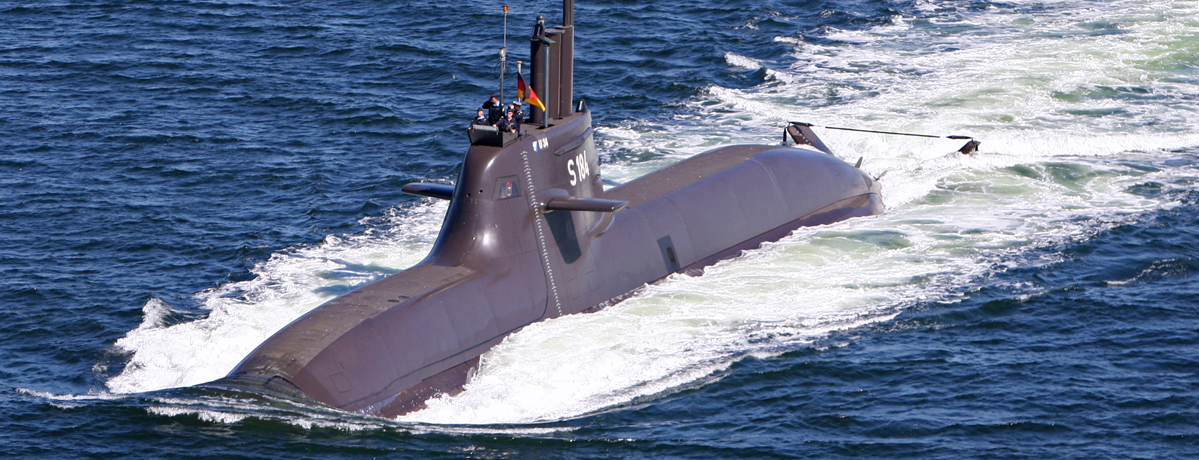This outdoor photograph captures a gunmetal gray submarine breaching out of the dark blue ocean, angling diagonally from left to right. The submarine is partially submerged, with water ripples and a foamy white wake marking its recent surfacing. On its side, the markings "S" and "182" can be seen. At the top on the observation deck, two figures are visible, accompanied by a colorful flag displaying shades of blue, orange, and yellow. The scene is bathed in sunlight, illuminating the still, vast expanse of the ocean.